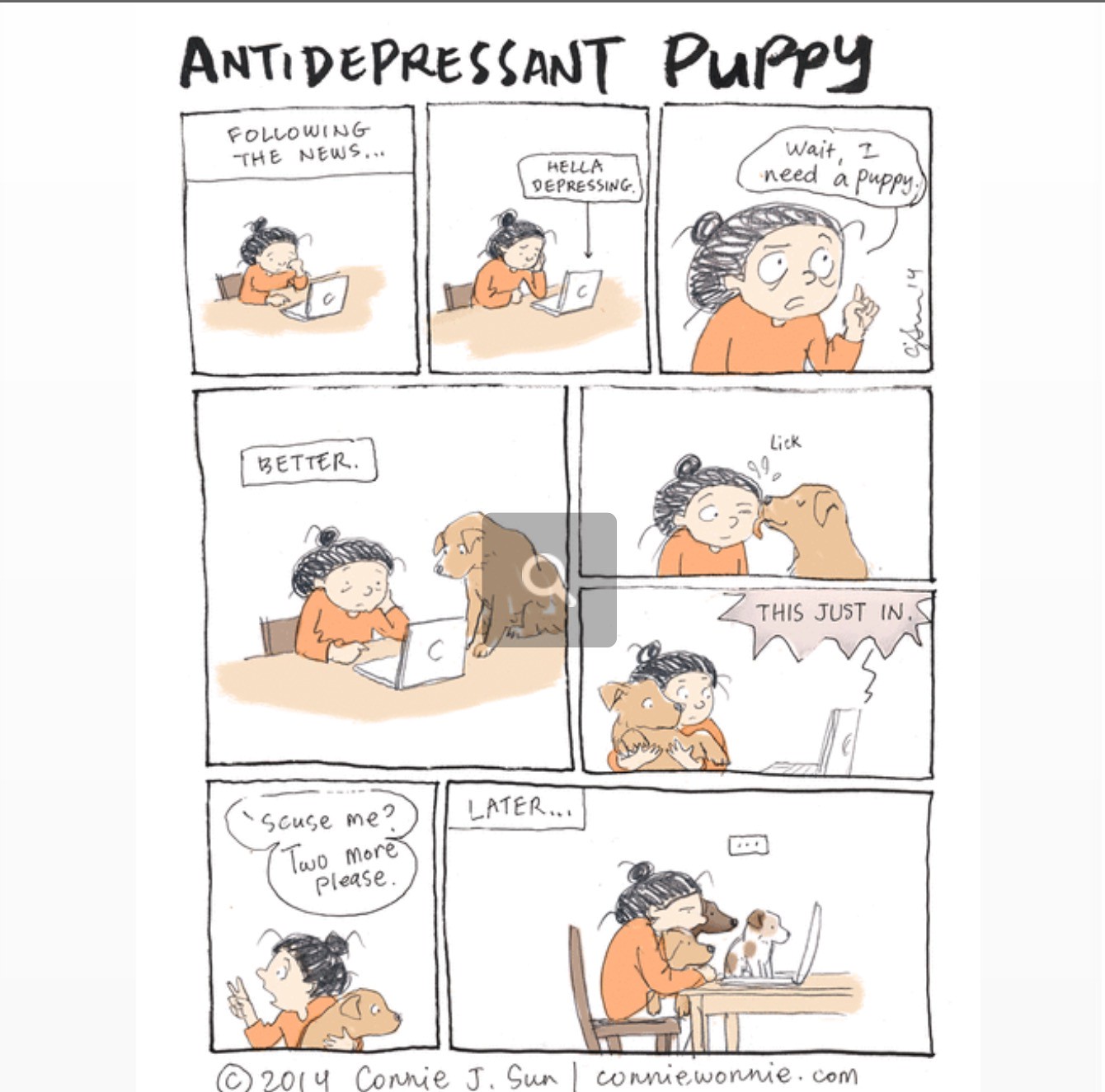The comic strip, titled "Anti-Depressant Puppy" by Connie J. Sun, features a sequence of panels that vividly depict a character's reaction to distressing news. The comic begins with a person looking disheartened while following the news on their laptop, captioned "Following the news... hella depressing." In the next panel, the character has an epiphany and declares, "Wait, I need a puppy." This is followed by a scene where the individual looks noticeably better as a puppy licks their face. However, as new, alarming headlines appear on the computer screen with a “This just in,” the character clutches the puppy desperately and exclaims, "Excuse me, two more please." The final scene shows the person, now surrounded by three comforting puppies, watching the news on the laptop, trying to find solace. This comic was created in 2014 by Connie J. Sun, and her work can be found at ConnieWani.com.